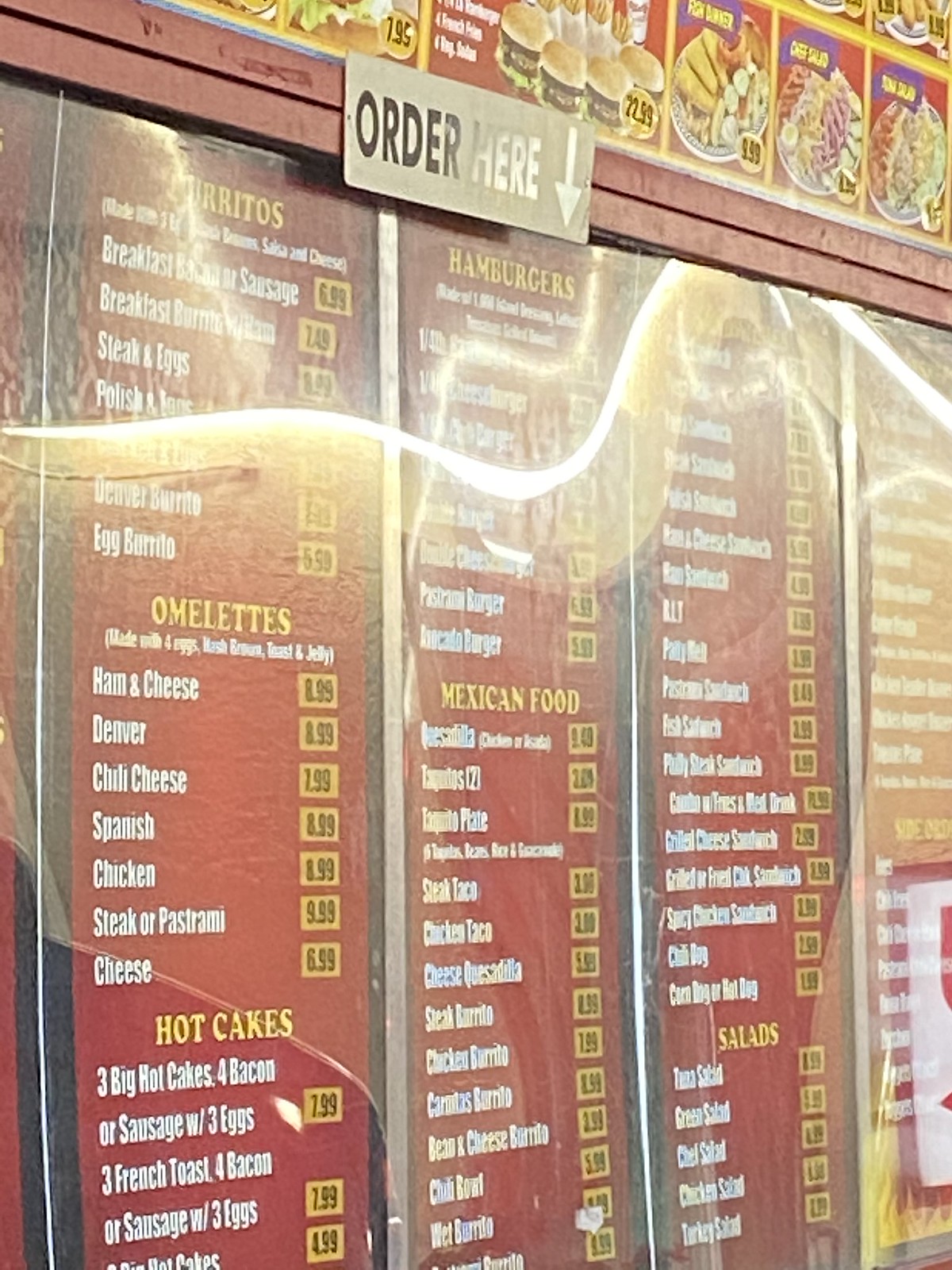This photograph captures a drive-thru menu with a red-bordered frame. Prominently displayed in the foreground is a black sign reading "Order Here" with a downward-pointing arrow. Above it, a red sign features yellow cubes adorned with images of various foods. The menu itself is somewhat obscured by a glaring yellow, wave-patterned line of light that makes parts of it difficult to read. 

The menu categories listed include Burritos, Hamburgers, Omelets, Mexican Food, Hot Cakes, Salads, and Side Orders. The text for the items is white, while the prices are highlighted in yellow boxes with black print on a red background.

Under the Omelet category on the left-hand side, the listed items are Ham and Cheese, Denver, Chili Cheese, Spanish, Chicken, Steak, and Pastrami and Cheese. The Hot Cakes section offers items like Three Hot Cakes, Four Bacon or Sausage with Eggs, Three French Toast, and Four Bacon or Sausage with Eggs, with prices ranging from $4.99 to $9.99. 

The Mexican Food category, though partially illegible due to the glare, includes items such as Quesadilla, Taquitos, Taquito Plate, Steak Taco, Chicken Taco, Chicken Quesadilla, Steak Burrito, Chicken Burrito, Carnitas Burrito, Bean and Cheese Burrito, Chili Bowl, and Wet Burrito.